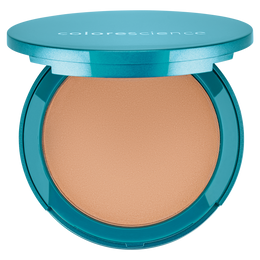The image features a product photo against an entirely white background, showcasing an open makeup container. The container consists of a teal-colored base and a matching solid teal top, which is positioned perpendicularly to the base. The makeup inside is a smooth, medium to dark tan shade, indicating it could be a foundation or concealer. The container is from the brand "Color Science," as indicated by the white text on the top, which is partially readable due to the angle. The teal packaging has a shiny finish, and the product remains unused.